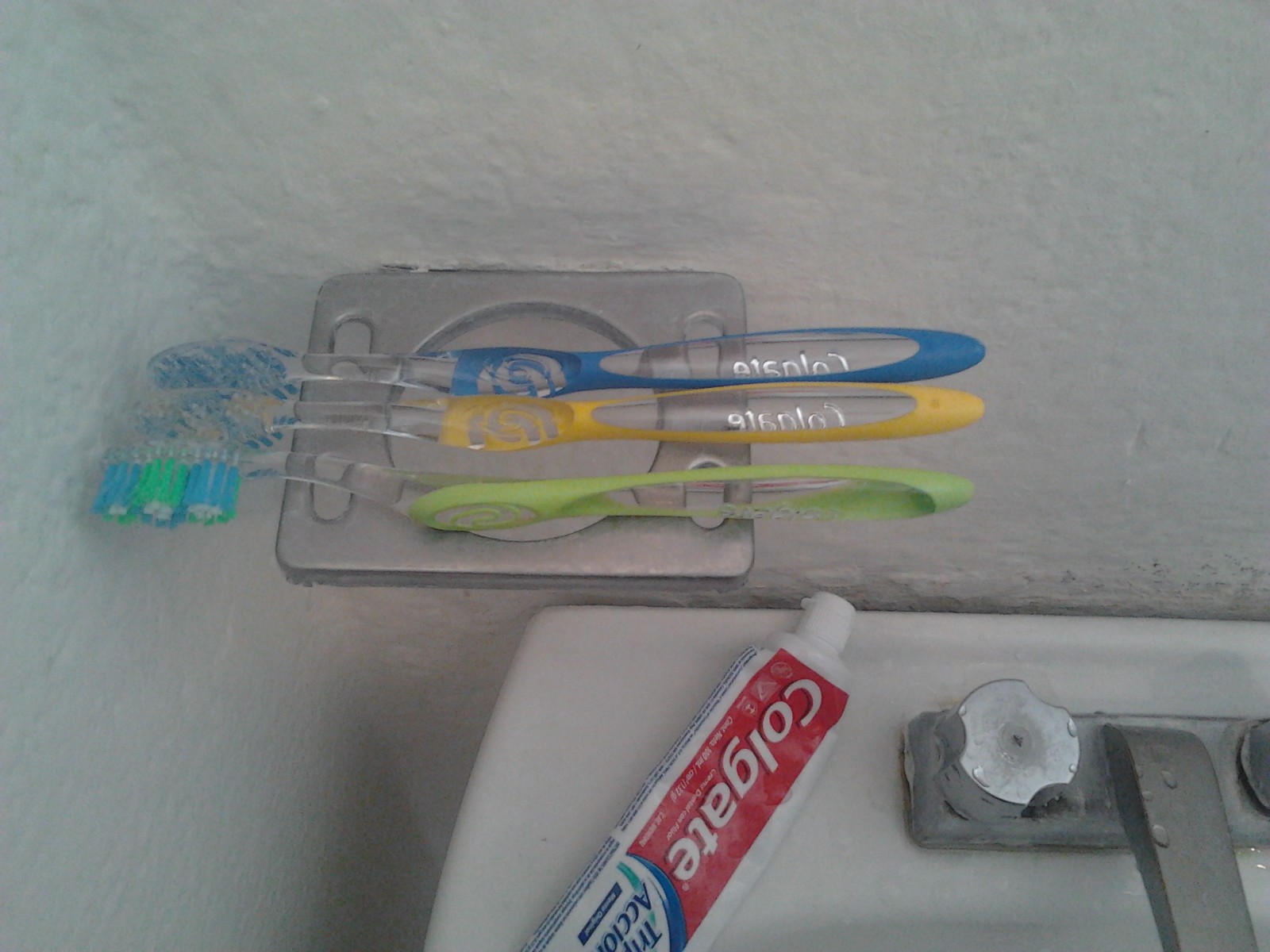The image depicts a partially visible porcelain bathroom sink mounted directly to a rough, unpainted white plaster wall. The sink features a silver faucet with a round white-topped knob and lacks an extended sink top. On the left side of the sink is a red, white, and blue tube of Colgate toothpaste with its cap on, labeled "Triple Action," appearing about 80% to 90% used. Above the sink, a brushed stainless steel holder, designed for a cup and up to four toothbrushes, is mounted to the wall. However, the holder currently has three Colgate toothbrushes laid sideways across it instead of being placed in their respective slots. These toothbrushes have clear handles with various colors: light green, yellowish-orange, and blue. The corresponding bristles are a mix of white, blue, and green.